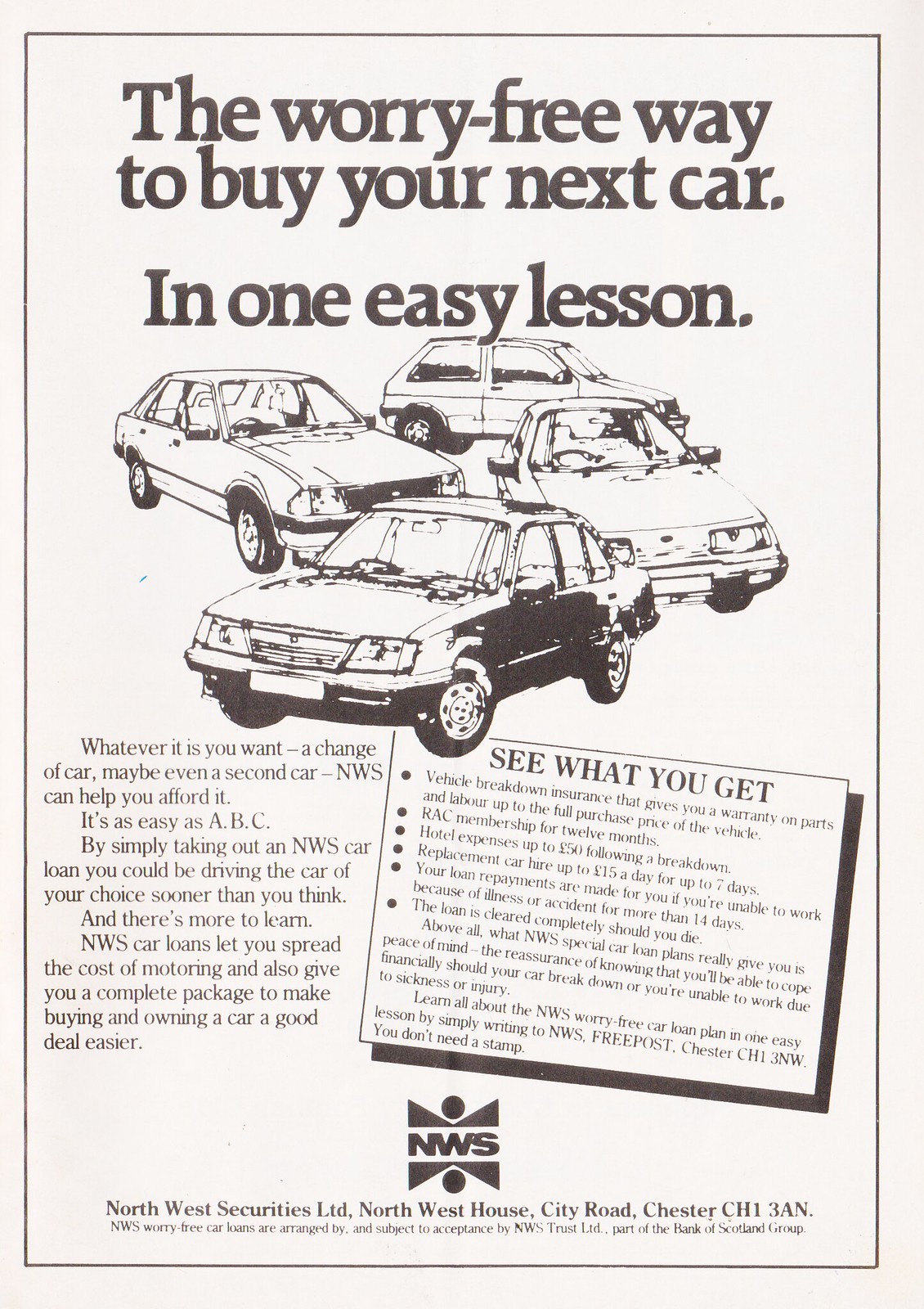This black-and-white advertisement appears in an old British football magazine, promoting the NWS Worry-Free Car Loan Plan. At the top, bold text declares, "The worry-free way to buy your next car in one easy lesson." Below this, there are black-and-white sketches of four different sedans, reflecting the style of cars from the time. Following the illustrations is a detailed chunk of text explaining how NWS can help you afford a new car, whether it's a change or an additional vehicle, emphasizing the simplicity of taking out an NWS car loan.

The text elaborates that by taking out a loan, you could be driving the car of your choice sooner than expected. NWS car loans allow you to spread the cost of motoring and offer a complete package to make buying and owning a car easier. To the right of the main text, there is a bullet-pointed list of perks included with the loan: vehicle breakdown insurance with part and labor warranties up to the car's full purchase price, 12-month RAC membership, hotel expenses up to £50 following a breakdown, car hire up to £15 a day for up to 7 days, illness or accident repayment coverage after 14 days, and loan clearance in the event of death. These benefits promise peace of mind, ensuring financial stability if the car breaks down or if the owner is unable to work due to illness or injury.

At the bottom of the ad, readers are encouraged to learn more by writing to NWS Free Post Chester CH13NW, with no stamp required. Additionally, it provides the detailed address of NWS Northwest Securities Ltd: Northwest House, City Road, Chester, CH13AN. The ad notes that these car loans are organized by and subject to acceptance by NWS Trust Ltd, part of the Bank of Scotland Group. The stark black text against a white background and the vintage car illustrations give this ad a classic, trustworthy feel.